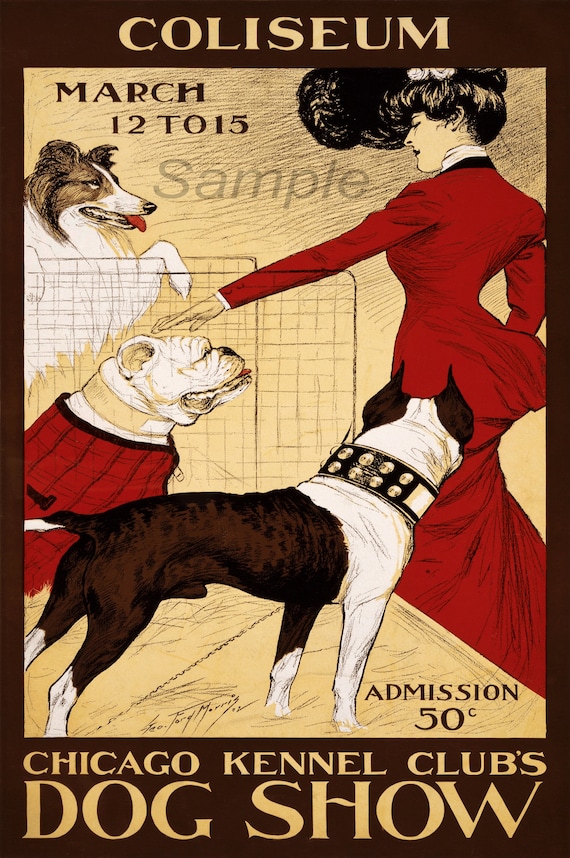This ornate, old-style poster promotes the Chicago Kennel Club's Dog Show held at the Coliseum from March 12th to 15th, with an admission fee of 50 cents. The poster, displaying a watermark with the word "Sample", features a central image set against a yellow rectangular background. In this depiction, a woman dressed in a long, 1920s-1930s era red dress with a puffy skirt, black undershirt, and her dark hair in an elaborate updo, stands on a wooden stage. She extends her hand to pet a white English Bulldog adorned with a red sweater and black accents. Flanking them on the stage are a Border Collie at the top, mostly white with brown patches around its eyes, ears, and face, and another Bulldog to the right, distinguished by its thick, spiked metal collar, chocolate brown ears, and a mix of brown and white fur. A reddish-brown border frames the bottom, highlighting "Chicago Kennel Club's Dog Show" in larger, prominent font. The detailed illustration captures the well-groomed nature of the dogs and the elegance of the event.